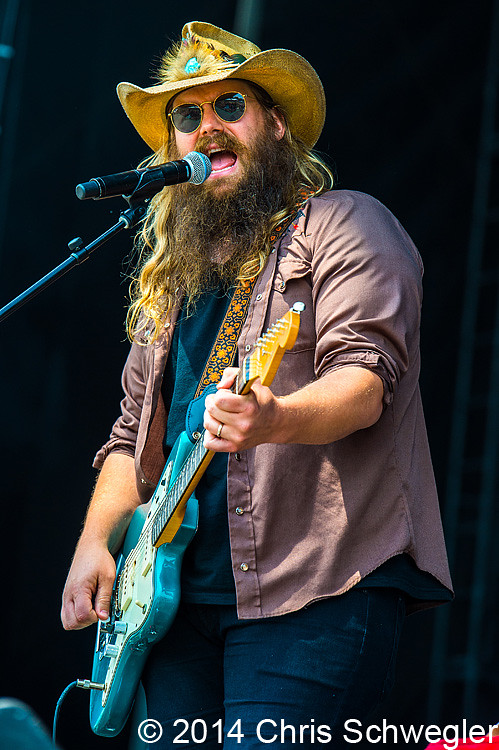The image features musician Chris Stapleton holding a seafoam blue electric guitar with a white front, plugged into an amp. Positioned center stage, Chris is poised with his guitar at crotch level, his left hand gripping the fretboard and his right hand playing the strings. A cordless microphone on a stand is placed right next to his mouth, indicating he's in the middle of a performance. He is wearing a very ornamental cowboy hat, sunglasses, a gray long-sleeved sport shirt with rolled-up sleeves, and a blue t-shirt underneath. His long hair and beard flow down below his shoulders. He also sports an intricately designed guitar strap. The setting appears to be an outdoor concert, with a darkened background highlighting his presence on stage. In the lower right corner of the image, the text reads "Copyright 2014, Chris Schweigler." The color palette includes the turquoise blue of the guitar, the brass color of its shaft, his beige skin, the light red shirt that appears pinkish, and the ornamental details of his attire.